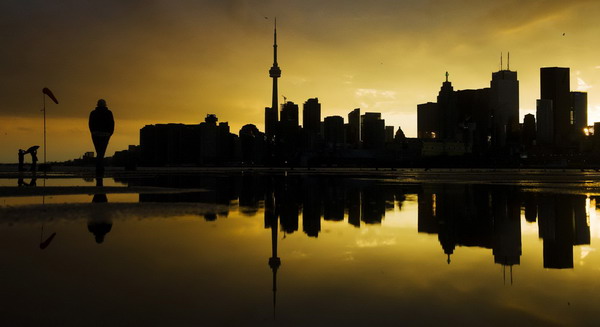This photograph captures a serene seascape at dawn, featuring a silhouetted skyline that is likely Toronto, identified by the presence of the iconic CN Tower. The image is taken in landscape orientation, placing the tranquil water in the foreground, with the perfectly flat and shiny sand suggesting waves recently washed over it. The horizon reveals a large city skyline with towering skyscrapers, all mirrored flawlessly in the calm water below. The sky showcases a stunning gradient from black to various darker shades of yellow, indicating the sun is just below the horizon, casting a glowing light behind the buildings. Off to the left-hand side, there is a silhouette of a person walking, accompanied by a pole with a windsock. Further in the background on the left, a couple more people can be seen, adding to the peaceful, early morning ambiance of this picturesque urban landscape.